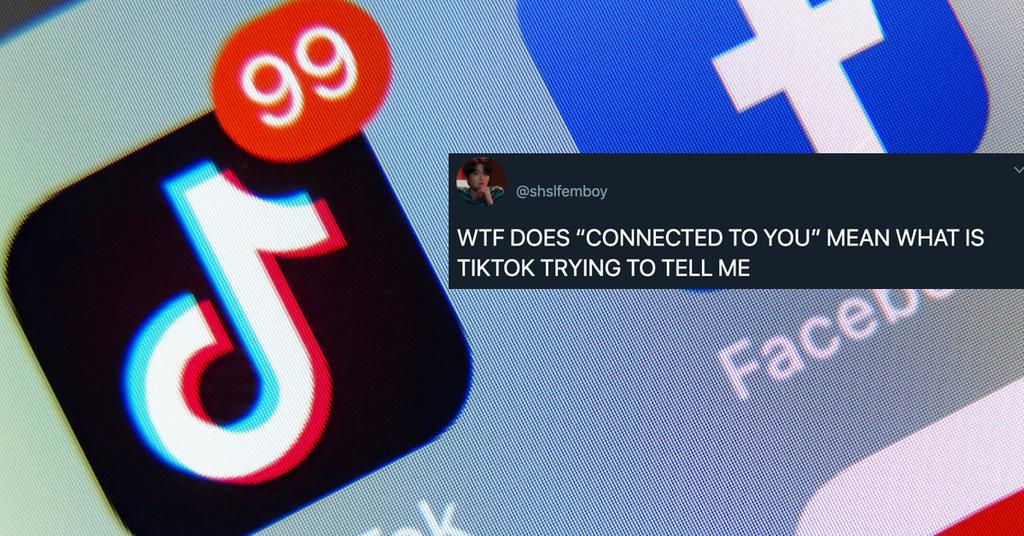The image primarily features a close-up shot of a pixelated phone screen, taken at an angle. On the left side of the screen is the recognizable TikTok logo, accompanied by the letter 'K' indicating the app's name. A red notification badge with the number '99' in white text is prominently displayed on the TikTok icon.

To the right of the TikTok icon, the partial Facebook logo is visible. While the top part of the Facebook icon is obscured and slightly cut off, it remains identifiable. Beneath the logo, part of the word "Facebook" can be seen, showing "face" clearly, followed by a 'B' and the beginning of an 'O'.

Overlaying this section of the screen is a black rectangle. In the top left corner of this rectangle, there is a small circle containing a dark, indistinguishable photo of a person. Next to the circle, the text "@SHSLFEMBOY" is present. The rectangle also contains a white, all-capitalized text against the black background that reads, "WTF DOES 'CONNECTED TO YOU' MEAN? WHAT IS TIKTOK TRYING TO TELL ME?"

In the bottom right corner of the image, part of another icon is visible, featuring a white border with some red beneath it. However, the partial view makes it impossible to identify the icon with certainty.